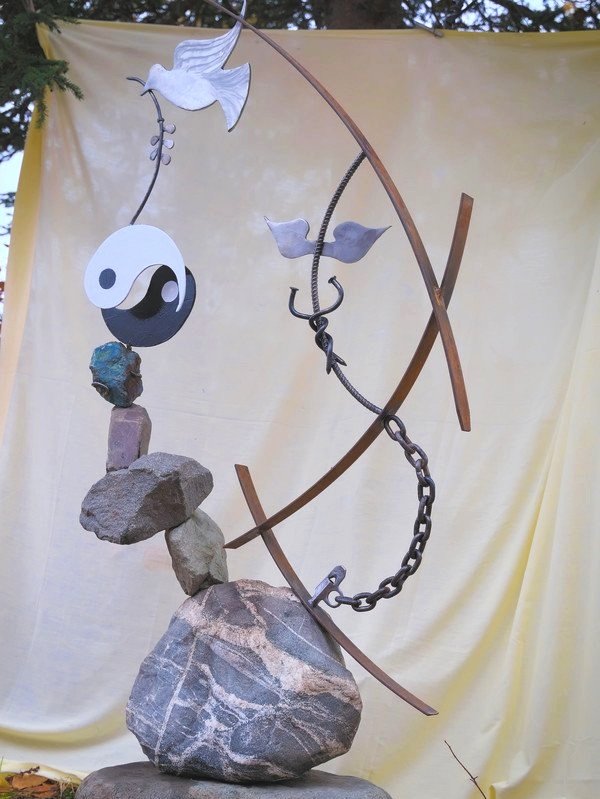The image portrays an intricate art piece situated against a yellow backdrop that highlights its details without distraction. The centerpiece of the art is a stack of gray and white marbled stones, seemingly balanced at improbable angles, suggesting they may be glued together. At the top of the stone stack rests a black and white yin and yang symbol, from which an olive branch sprig and a white dove extend outward. Descending from the largest bottom stone, a chain adorns the sculpture, featuring red metallic bands and silver blades. The entire scene is framed by a gray-colored background, with hints of dark brown anchors or chains linking various elements. The art piece subtly integrates complex details, including additional gold metal pieces and an anchor with a ribbon, creating a harmonious blend of natural and metallic elements.